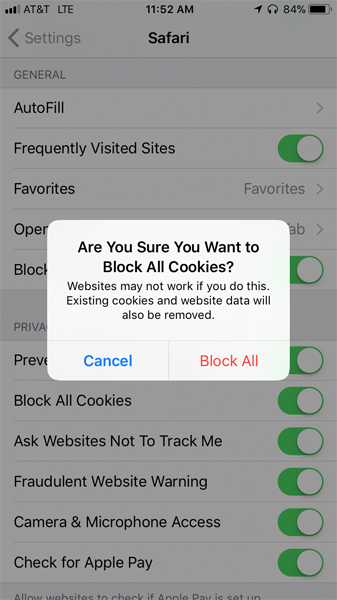This image is a detailed screenshot from an iPhone, focusing on a prominent prompt about cookies in the Safari settings. The screen is partially dimmed to emphasize the prompt, which is a white, semi-rectangular box with curved edges and black text. The message reads: "Are you sure you want to block all cookies? Websites may not work if you do this. Existing cookies and website data will also be removed." Below this message are two options for user action: "Keep" in blue text and "Block All" in red text.

In the background, the image reveals the settings interface of the iPhone, specifically in the Safari section, as indicated by "Settings" and "Safari" at the top of the screen. The dimmed interface shows a list of browser options, including "Block All Cookies," "Ask Websites Not to Track Me," "Fraudulent Website Warning," and permissions for camera and phone access, among others. The screenshot captures the user experience of navigating privacy and security settings within Safari on an iPhone.